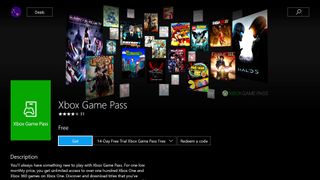The image appears to be a slightly blurry, small snapshot of an Xbox Game Pass interface, likely captured from either a tablet held in landscape mode or a laptop. The background is predominantly black, with various UI elements scattered across the screen. In the upper left-hand corner, there's a barely readable, small purple circle accompanied by an adjacent button. A search icon is situated in the upper right-hand corner.

In the bottom left corner, the word "Description" is displayed in white text, below which lies a portrait-oriented green rectangle. Next to this rectangle, "Xbox Game Pass" is prominently mentioned. Above this, a visually striking, animated selection of game titles arches in a dynamic pattern, showcasing the variety and excitement of the available games. Toward the right, there's a blue box, presumably a purchasable button, indicating that this interface serves as a shopping platform for Xbox Game Pass, possibly on Xbox.com or a related purchasing site. The remaining parts of the image are predominantly black, with most text elements being too small to decipher.